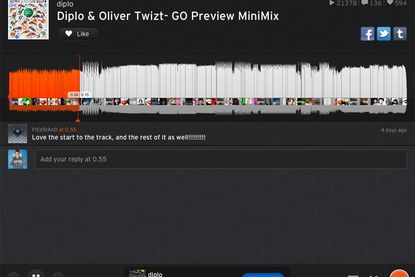This image depicts a website designed for desktop use, set against a black background that makes visibility challenging. The bottom part of the website is cut off, obscuring some icons. 

In the top left corner, there is a white box containing various elements, while a prominent blue-teal circle is centered at the top. The text "Diplo and Oliver Twizt - Go (Preview Mini Max)" appears in white font; note that "Twizt" is spelled T-W-I-Z-T. Below this text is a black button with the word "like" and a white heart, indicating the item has been liked.

On the right side, under the like button, there are icons for Facebook and two versions of Twitter, possibly representing different Twitter accounts or versions. 

Beneath these social media icons, a graph that likely displays sound waves from a musical performance is visible. The initial third of the graph is red, transitioning to an antique white for the remainder. 

Following the graph, there are very small graphics in bars, representing each second of the song or visual element. Further down, there are two rows containing additional, unspecified elements.